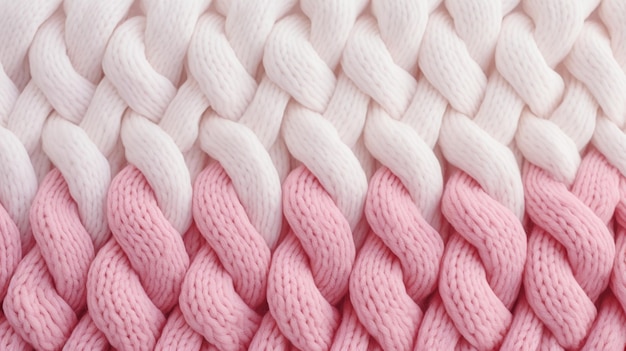This image features a close-up view of an intricately braided knitwork, possibly resembling a blanket or a quilt. The weave is composed of thick, noodle-shaped strands that evoke the texture of shoestrings. These strands are tightly knit into a detailed pattern of braids, with larger strings interlacing to create a cohesive and robust fabric. The top half of the image showcases a white or very light pastel pink color, while the bottom half transitions into a much darker pink hue. The woven pattern appears in repetitive columns, suggesting a complex and structured design that could potentially be part of a larger object such as a basket or cozy sweater, characterized by its warmth and comfort.